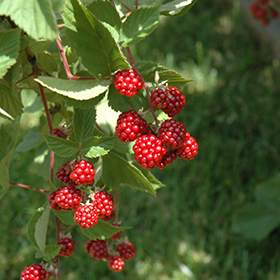This detailed photograph captures multiple clusters of ripe red raspberries thriving on their thorny, light-red vines. The focal point is the vibrant raspberries with their lush light-green leaves, creating a stark contrast against the blurred greenery in the background, which appears to be grass or bushy foliage under sunlight. There are at least four clusters, each with varying quantities of berries—some clusters comprising around seven raspberries, while others contain about five or even up to eight. The image is bright, with the sunlight casting subtle shadows and making the raspberries appear even juicier and ready for picking. The background's deliberate blur enhances the focus on these succulent fruits, emphasizing their rich color and ripe readiness against the leafy, sunlit environment.